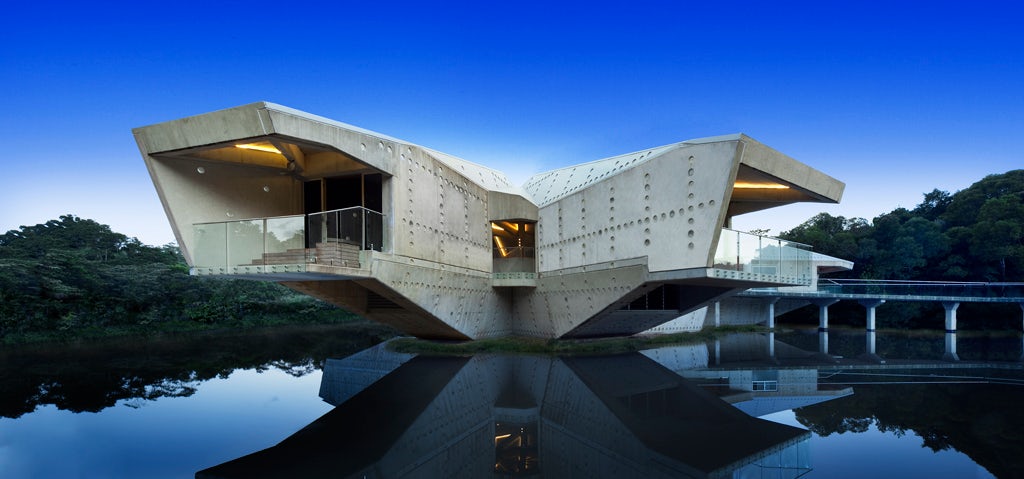The image showcases a contemporary, angular building with an intriguing design, possibly a digitally rendered concept. The structure is composed of gray concrete or metal panels adorned with grid-like patterns of small circular bolts. This unique building is split into two main parts forming an inverted V-shape, each part extending outward to the left and right with glass-fenced balconies above a serene body of bright blue water. The water is so still that it reflects the building's image perfectly. Connecting the two extensions, a small central deck area also features glass railings. Illuminated by orange lights installed on the deck ceilings, the building exudes a warm glow as if captured during dusk against a backdrop of a dark blue, cloudless sky. Surrounding the building, there are green trees contributing to a natural ambiance, and a bridge on the right, which also has a glass railing, leads to what appears to be a parking space. The combination of innovative architecture and picturesque natural elements suggests that this could be a travel or industry photograph.